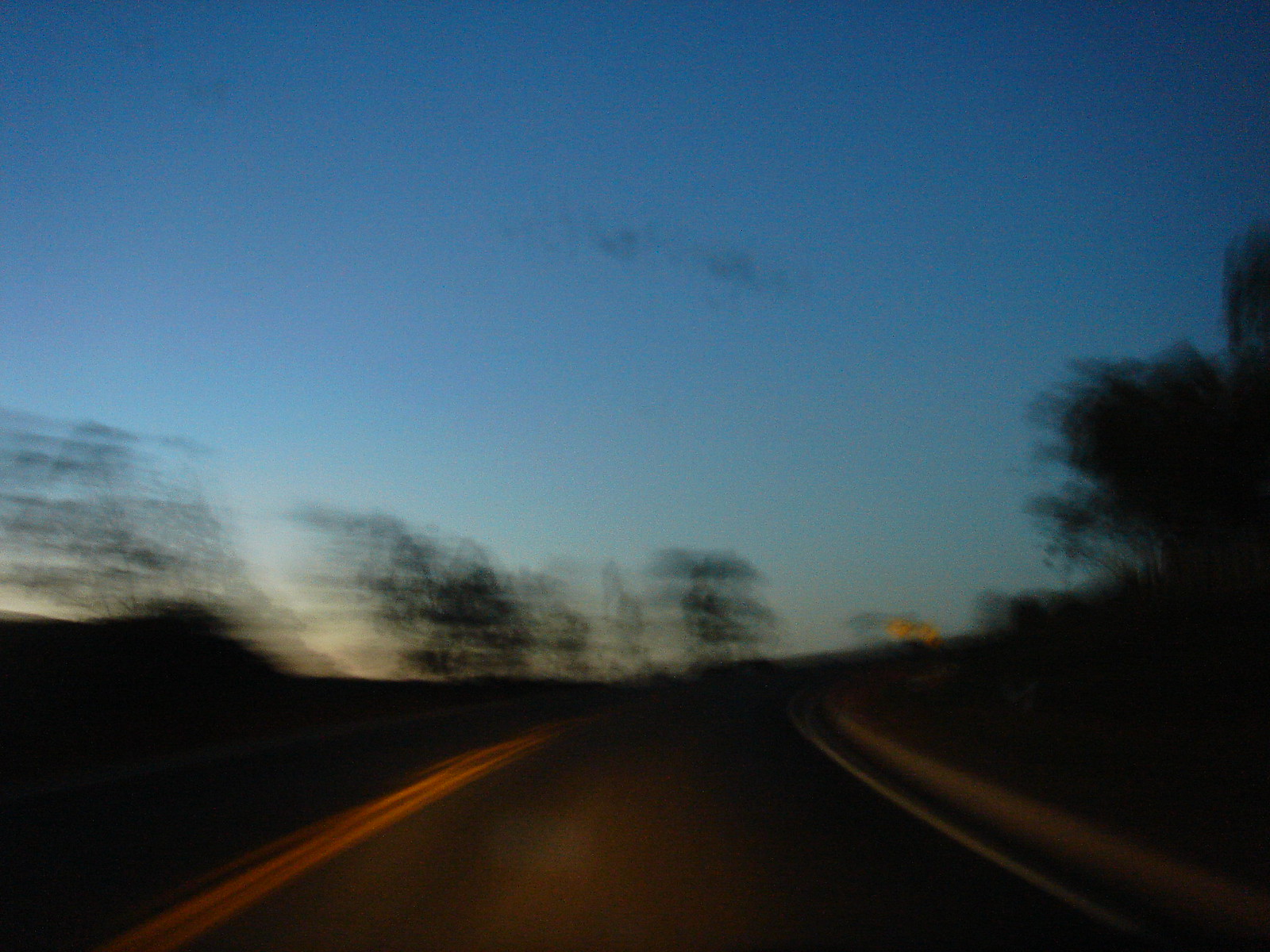In this image, we see a blurry photograph of a winding street taken from inside a moving vehicle, likely a car. Captured either just before sunrise or just after sunset, the sky presents a dark blue hue, gradually fading to a lighter shade near the horizon, silhouetting the surrounding trees and bushes. The road curves gently to the right, marked by a double yellow line running down its center. Yellow road signs can be faintly seen ahead. Owing to the low light conditions and the movement of the vehicle, the scene appears indistinct and blurry, with the camera unable to sharply focus on the details, adding a sense of motion and dynamism to the picture. The photograph is devoid of any text.